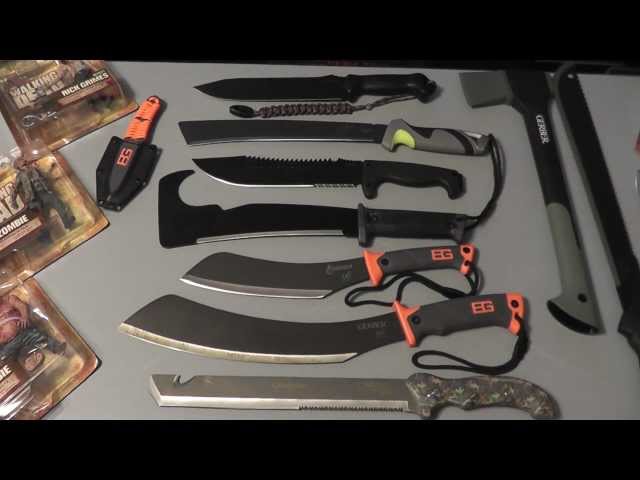The photograph showcases an array of seven hunting knives meticulously arranged on a gray, rubberized surface. These knives, with their sheaths removed, exhibit a variety of blade styles including serrated edges and one distinctive knife featuring a curved hook back. Their handles, in diverse colors and materials, contribute to their unique appearances. Positioned to the right of the knives are two additional bladed instruments: one resembling a fire axe with a gray and black handle, and another elongated, undefined tool. The image is letterboxed with black horizontal bars at the top and bottom, hinting that this might be a still from a video. 

On the left-hand side of the image are three packaged action figures from "The Walking Dead" series, prominently featured in their plastic blister packaging. These include characters like Rick Grimes and presumably a zombie, reflecting the show's theme of survival and weaponry. Nestled between the action figures and the hunting knives is a peculiar triangular black device made of plastic, adorned with a small orange strap. All these items rest on the gray surface, coming together to form a striking collection of weaponry and collectible memorabilia.